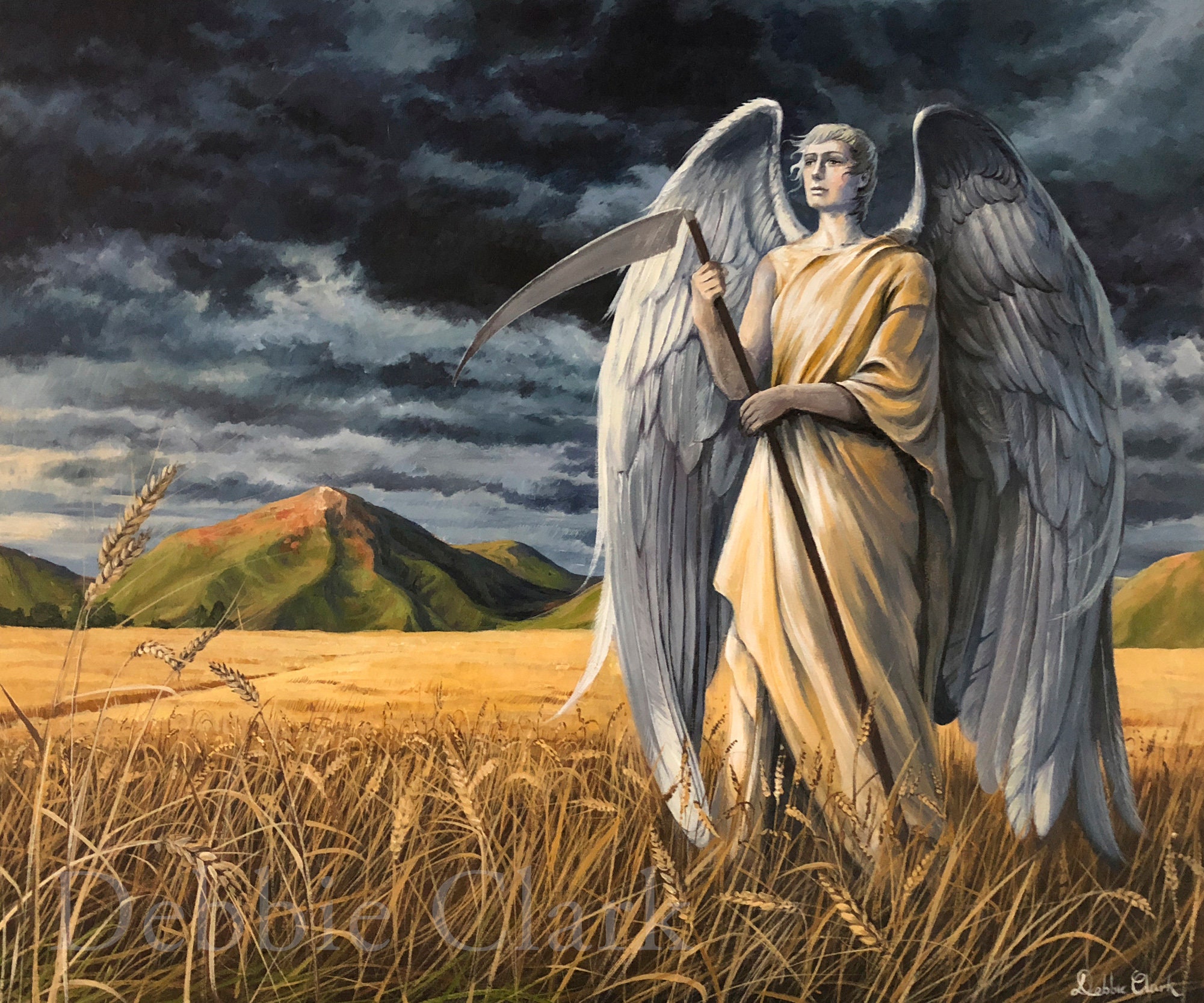This painting depicts an angel, likely Gabriel, standing solemnly in a golden wheat field under a foreboding sky filled with dark grey clouds. The wheat in the foreground is a vibrant yellow and tan, becoming more flat and faded towards the horizon where light green highlights trace the rocky or hillside areas. In the background, distant green mountains add depth to the scene, their tops tinged with brown and white under the ominous sky.

The angel dominates the right-hand side of the image, draped in a gold or off-white toga with one sleeve extending down the left arm while the right is bare. His massive, detailed white wings arch over and above his head, hinting at both his ethereal nature and protective stance. Gabriel stands with a worried expression, looking up and to the left, gripping the staff of a sickle or scythe—a tool symbolic of harvest and judgment.

The intricate details of the painting, which may be rendered in graphite or pencil, suggest a blend of ancient and contemporary styles. The entire image is darkening as the heavy clouds encroach, casting an increasingly menacing aura over the scene. In the lower right-hand corner, the artwork is signed by Debbie Clark, a name also faintly watermarked at the bottom, signaling the artist’s identity. The landscape and the angel together create a powerful visual narrative of impending change or judgment under a stormy sky.